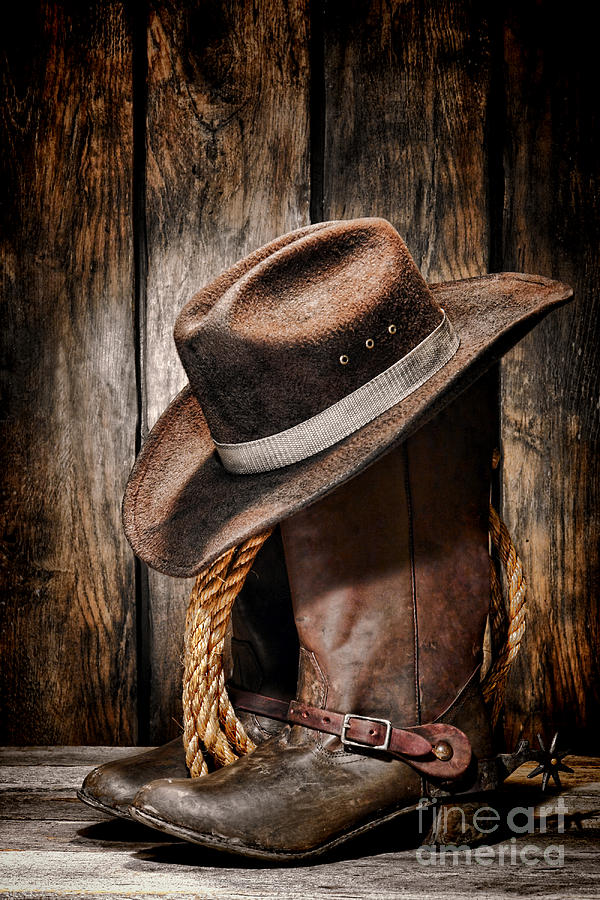This color photograph captures a striking scene that evokes the essence of the Old West. Central to the image are a pair of well-worn brown leather cowboy boots, adorned with silver-buckled spurs attached by a leather belt. Positioned between the boots is a light brown rope, artfully coiled and adding to the rustic charm. Atop the boots rests a brown suede cowboy hat, tipped forward and encircled by a gray band. The background features dark, aged wood with pronounced grain and black streaks, giving a barn-like atmosphere, while the boots stand on a contrasting gray wooden surface. In the bottom right corner, a semi-transparent white "Fine Art America" watermark can be seen, lending a touch of modernity to this timeless representation of cowboy life. The portrait orientation of the photograph further accentuates the vertical alignment of these iconic Western elements.